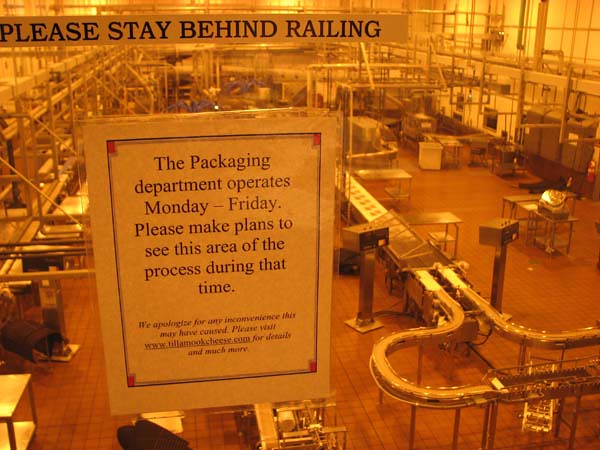This detailed photograph depicts the interior of a cheese factory's packaging department, viewed through a glass window. The image has a sepia or orange tint, possibly due to the window or photo quality. Prominently displayed on the glass window is a white laminated sign, bordered in black with red squares at each corner. The sign reads: "The packaging department operates Monday through Friday. Please make plans to see this area of the process during that time. We apologize for any inconveniences this may have caused. Please visit www.tillamookcheese.com for details and much more." Above the sign, a black-lettered label instructs, "Please stay behind railing," indicating safety precautions for potential tours. The factory floor, visible through the window, is densely populated with an array of machinery, metal tables, equipment, and pipes, as well as blue mechanical arms in the distance. Despite the extensive setup, no personnel are present, suggesting the photo was taken outside of regular operating hours.